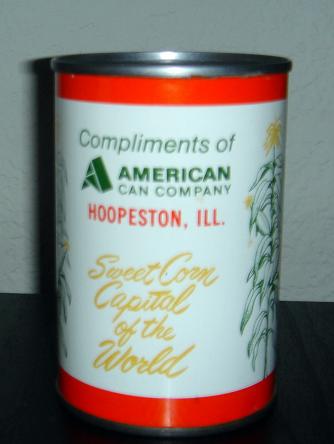The image depicts a slightly blurry, close-up photograph of a canned food product, specifically a can of sweet corn. The can appears to be approximately 13 ounces and features silver metal rims at the top and bottom. The label is predominantly white with narrow red stripes bordering the top and bottom edges. 

In the center of the label, it reads "Compliments of American Can Company" in green text at the top, followed by "Hoopston, Illinois" in red text beneath it. On the lower half of the label, "Sweet Corn, Capital of the World" is written in yellow cursive text. The label also includes outline drawings of green corn stalks with yellow tassels on the left and right sides, though these are partially obscured as they are located near the edges of the can.

The can is positioned on a black, smooth surface in front of a textured gray wall. A shadow of the can falls slightly to the left on the wall behind it.